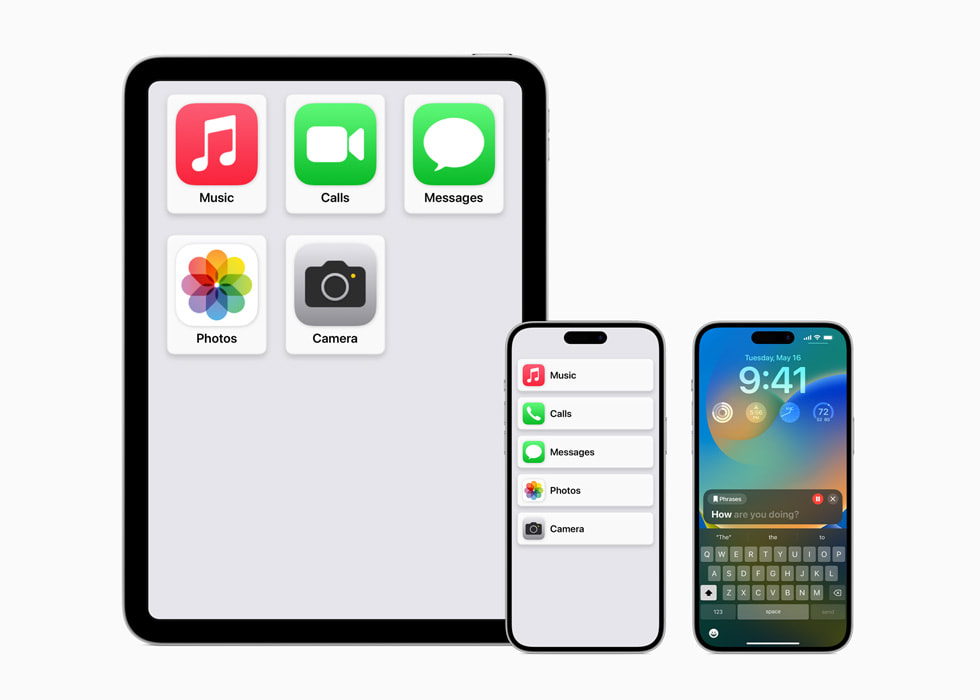In this image, set against a white background, an iPad and two iPhones are standing adjacent to each other. The iPad is positioned to the left and slightly overlaps with the first iPhone, which is also partially obscuring the second iPhone to its right. The iPad screen displays a simplified operating system with significantly enlarged icons for the Music, Calls, Messages, Photos, and Camera apps, designed for enhanced accessibility. Similarly, the first iPhone showcases a home screen with large, user-friendly icons arranged in a widget-style format, with apps like Music, Calls, Messages, Photos, and Camera taking up substantial space for ease of use. The second iPhone displays a lock screen featuring the date Tuesday, May 16th, 9:41 AM, along with various widgets for tracking movement and weather. It also shows an active text message conversation, responding to a message while on the lock screen. This setup appears tailored for older adults or individuals with visibility challenges, offering larger text and icons to improve usability.